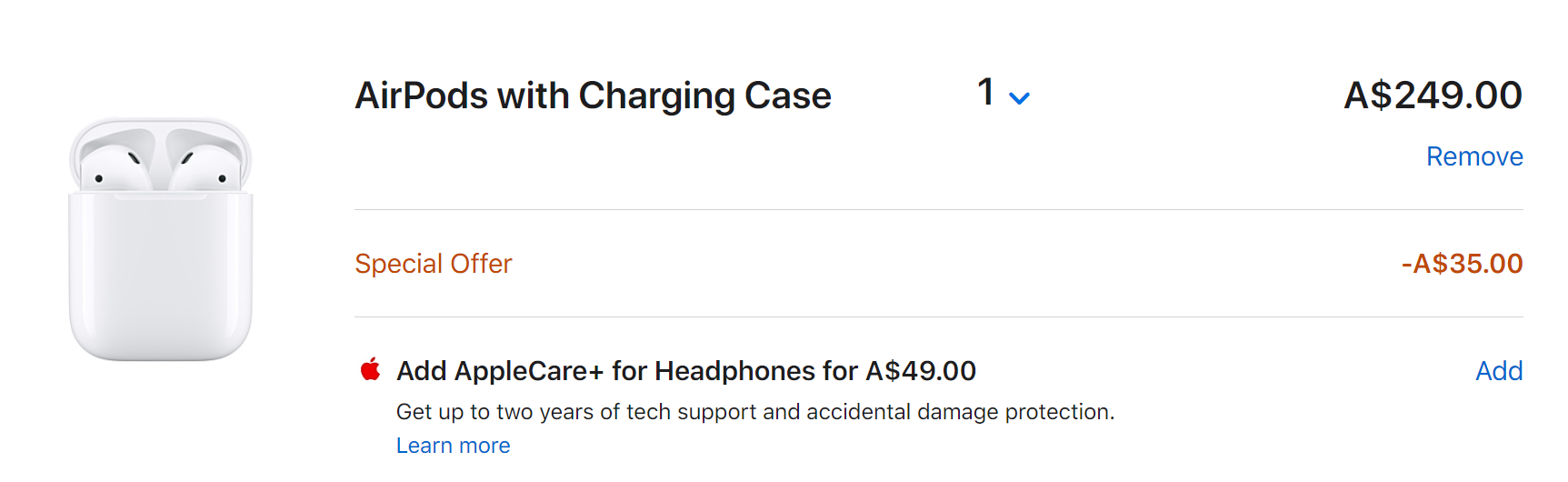The image appears to show a section of an e-commerce website where a user is reviewing their potential purchase of Apple AirPods with a charging case. The product in question is a pair of white AirPods, accompanied by a matching white charging case. The text "AirPods with Charging Case" is prominently displayed in black on a clean white background in the upper-right section of the image. The current quantity is set to one, with an option to adjust this through a drop-down menu.

The displayed price is $249, and there is an indication that the item can be removed from what appears to be a shopping cart or basket. Beneath the item description, a "Special Offer" label is highlighted in red, indicating a discount of $35—though it’s unclear whether this discount is already included in the displayed price or is an additional reduction.

Additionally, there's an option to add AppleCare+ for headphones at an additional cost of $49. This option is available via a blue button and offers up to two years of technical support and accidental damage protection. Further information about AppleCare+ can be accessed as indicated in the description.

Overall, the layout is user-friendly with clear labeling and options for modifying the order and adding warranty coverage, ensuring a straightforward and informative shopping experience.